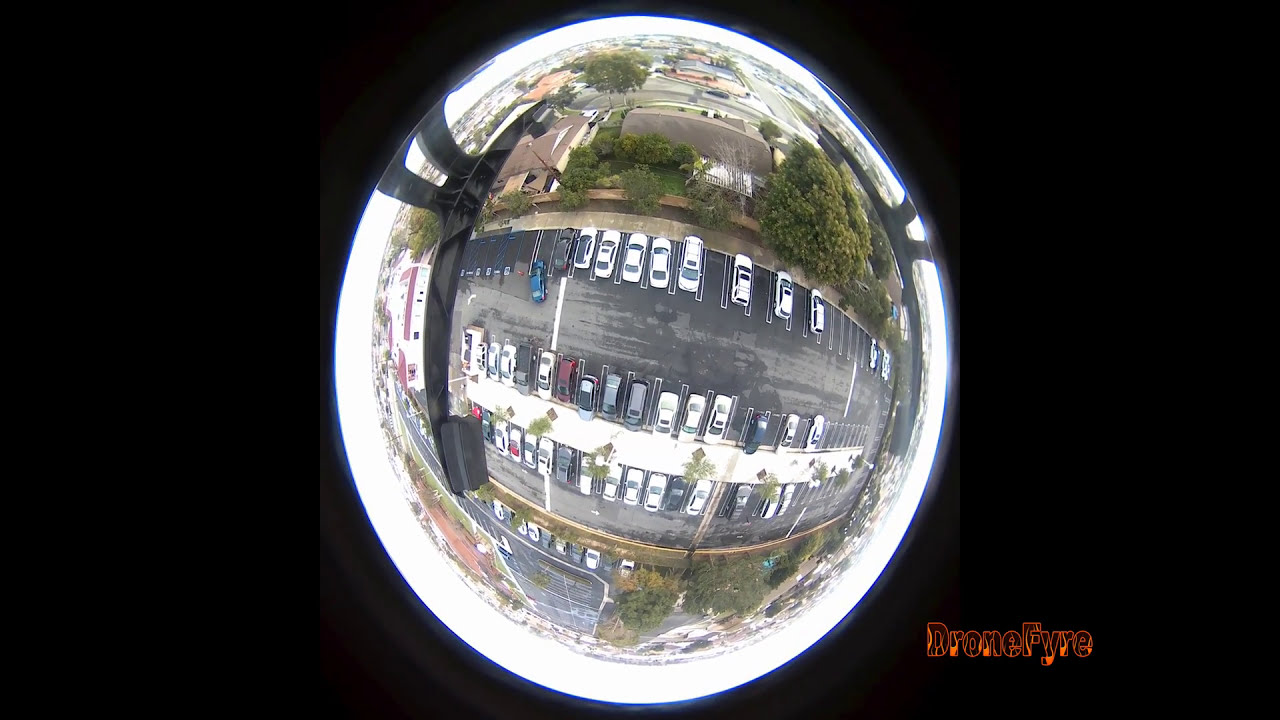This is a detailed bird's-eye view of a parking lot, captured from a drone hovering about 50 to 100 feet high. The image has a fisheye or convex effect, creating a circular distortion that becomes more pronounced towards the edges. Surrounding the circular image is a black background with blue and white concentric circles. In the bottom right corner, orange text with a flame effect spells out "DRONEF-Y-R-E." The parking lot, seen from above, is filled with various types of vehicles such as sedans, pickup trucks, SUVs, and notably, a maroon car and a blue car pulling out. The lot itself shows patches of wet and dry concrete, with white markings delineating the parking spaces. Trees and pathways run through the center, and surrounding the lot are various buildings and a mix of residential and urban features typical of an American neighborhood.